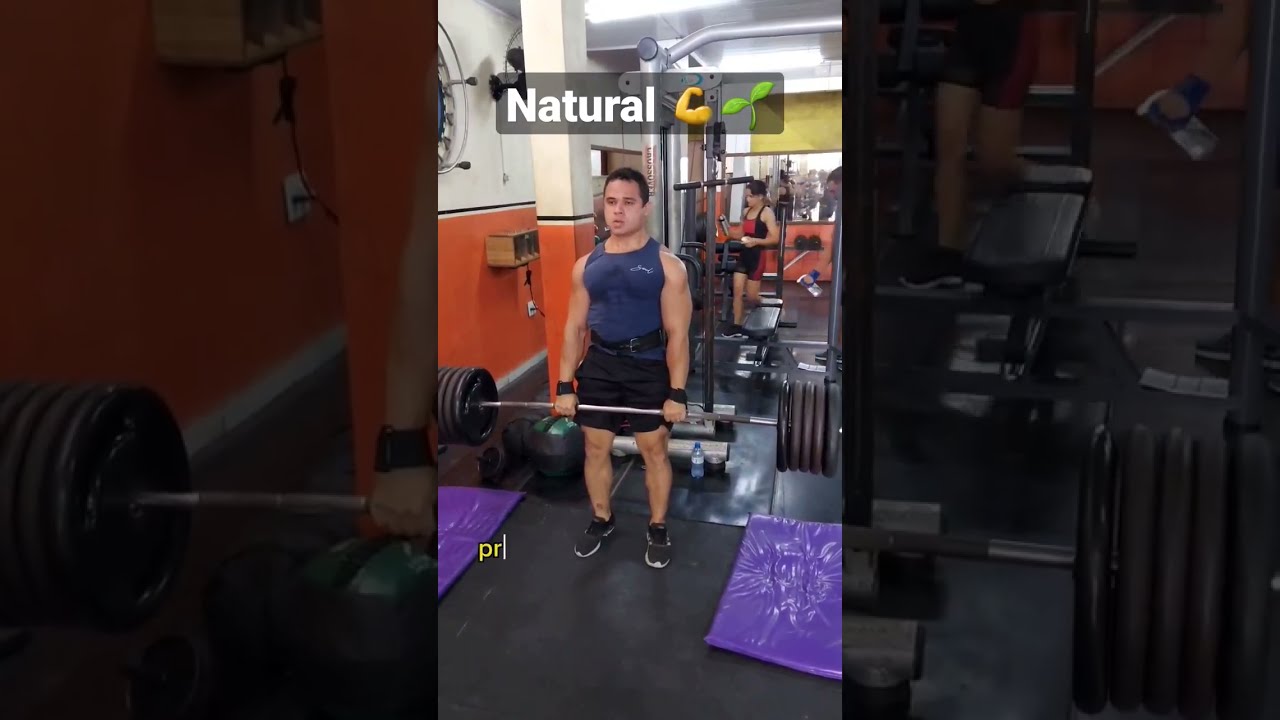The image is a screenshot from a social media post, likely from TikTok or Instagram, showcasing a man with light brown skin and short black hair lifting weights in a gym. He is performing deadlifts, holding a large barbell with five weights on each side. The man is dressed in a sleeveless blue tank top with white print, black shorts, black shoes, and black wristbands, and he is wearing a black weight lifting belt around his waist. The gym has distinctive red and white walls, though other sources describe parts as orange and white, with various workout machines and weights visible. Behind the man, a woman and another gym-goer can be seen working out. The black floor features a purple mat where the weights rest. The post includes a caption that reads "natural," accompanied by an emoji of a flexing arm and a two-leafed plant, displayed in a see-through rectangle towards the top. The overall composition of the image includes enlarged, darkened sections of the barbell on either side for effect.